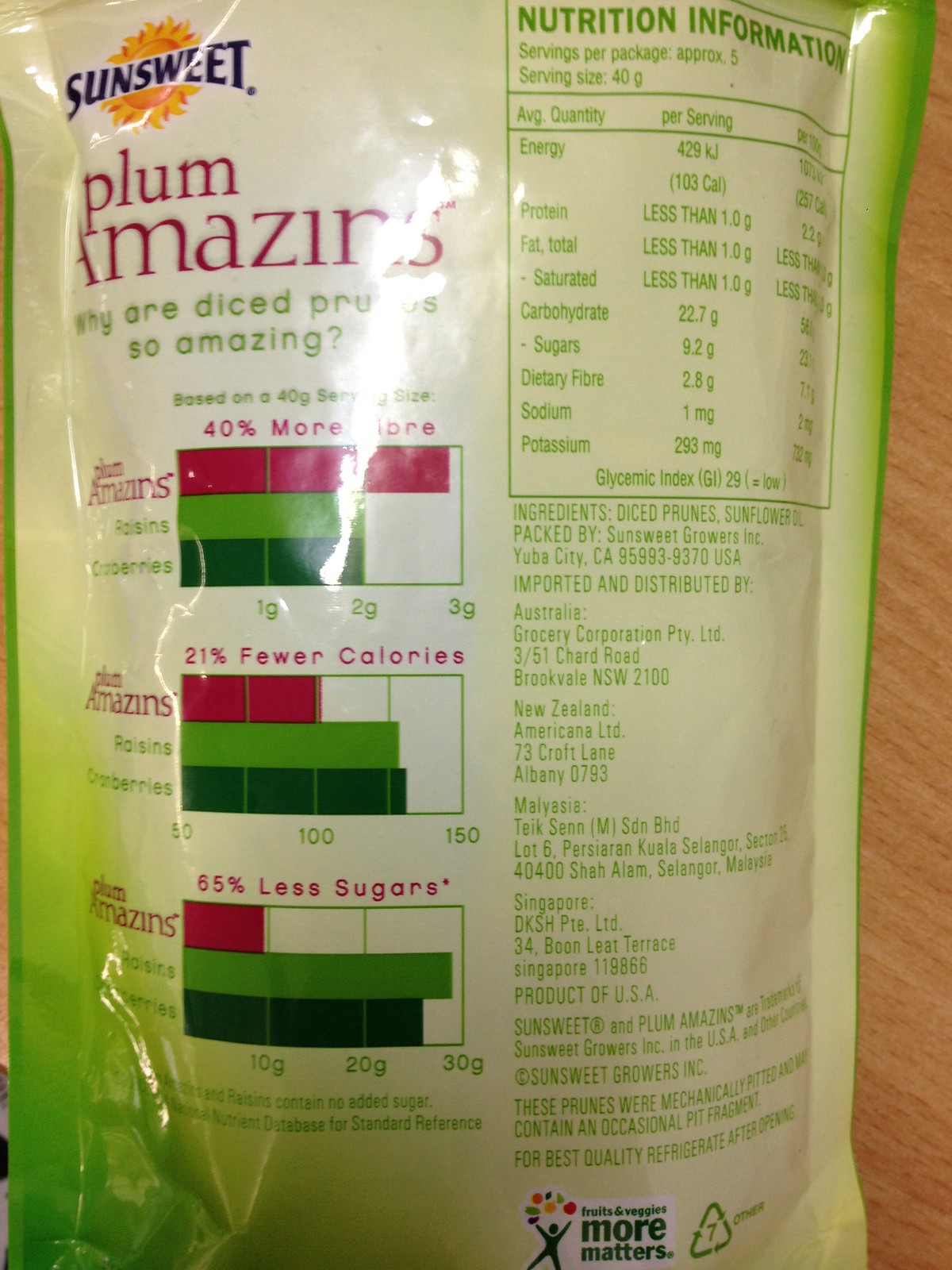This image is a zoomed-in shot of the back of a white and green bag of SunSweet plums, taken indoors. Prominently featured on the top left of the bag is an orangish sun logo with "Sunsweet" written in blue. Below the logo, in purple text, it reads "Plum Amazins" followed by the question, "Why are diced prunes so amazing?" Three bar charts are present, showcasing the nutritional benefits: 40% more fiber, 21% fewer calories, and 65% less sugar. The right-hand side of the image details the nutritional information, including energy (429 kJ), protein, total fat, saturated fat, carbohydrates, sugars, dietary fiber, sodium, and potassium. The middle portion of the right side lists the ingredients, mainly diced prunes with sunflower oil, and mentions that the product is packaged by SunSweet Growers in Yuba City, California, and distributed in regions such as Australia, New Zealand, Malaysia, and Singapore. At the very bottom, there’s a message that reads "more matters" accompanied by a stick figure with colorful dots above it.